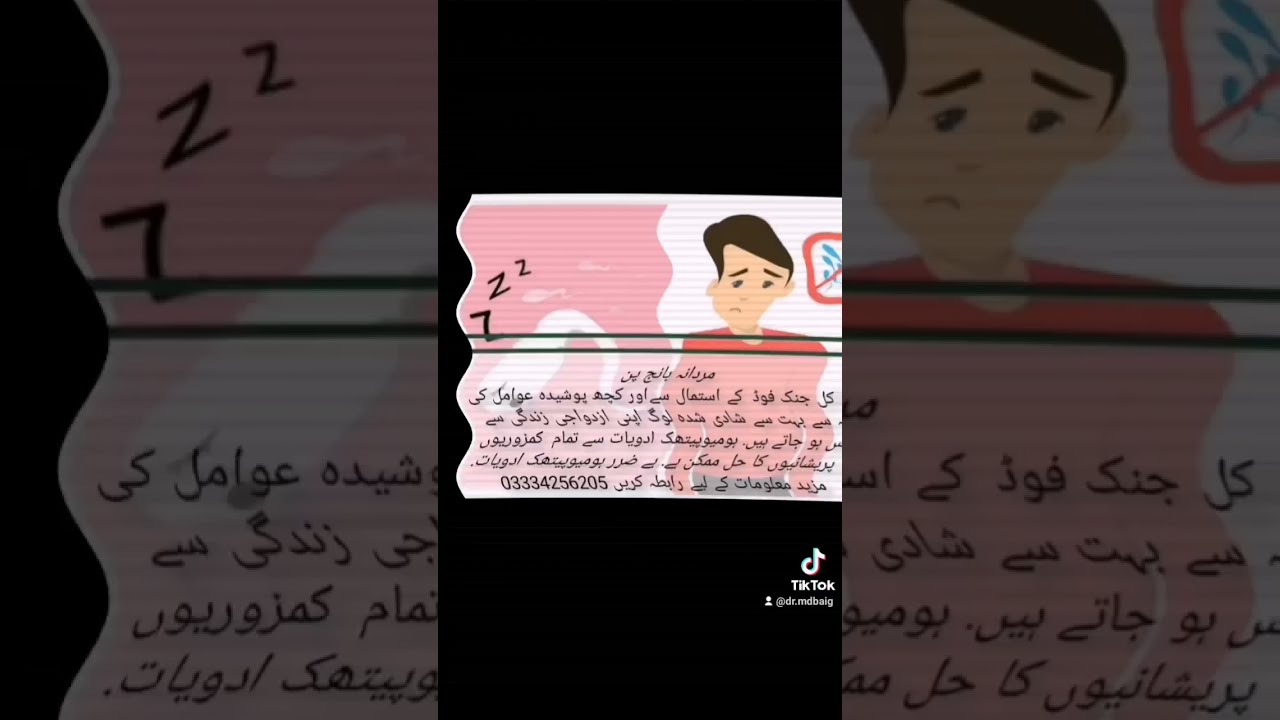This is a vertical phone screenshot from TikTok, featuring a prominently central image with a black rectangular background segmented into three vertical stripes. The central stripe contains a smaller, wavy-edged rectangle with a pink and white background. Inside this rectangle is a cartoon drawing of a sad-faced man in a pink shirt. The left side of this smaller rectangle has black "Z" figures against the pink background. Beneath the cartoon, there is a series of six lines of foreign cursive writing in black font. The outer two vertical segments of the image mirror the wavy rectangle but in darker, duller shades. At the bottom of the image, towards the right, sits the TikTok logo, indicating the image's origin from the platform. Additionally, a series of numbers—03334256205—appear at the bottom left of the image.